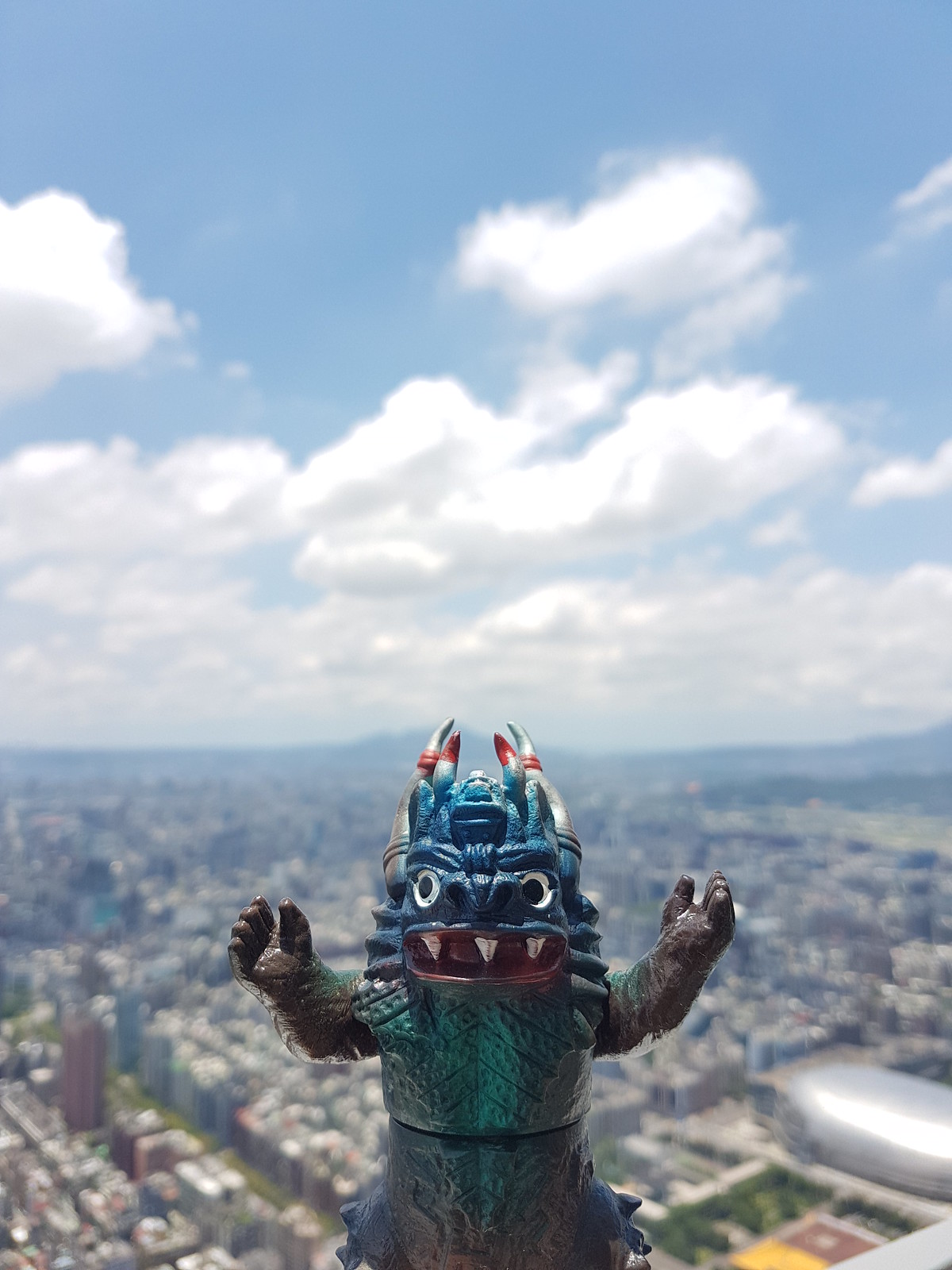In this striking image, we see a detailed plastic figurine held against an outdoor city backdrop. The figurine, resembling a Godzilla-like character or possibly a cultural deity, features a blue face with a red mouth and three prominent white teeth. It boasts spiked hair, horns tipped in red, white, and blue, and dark brown hands extended outward. The body is adorned in a blue suit of armor. In the distance, a sprawling cityscape with numerous skyscrapers is visible, set against a backdrop of majestic mountains. The sky above is a vibrant blue, punctuated by both white and gray clouds, with the sun casting a bright glow over the scene. This captivating composition seamlessly blends detailed foreground artistry with an expansive, scenic urban landscape.